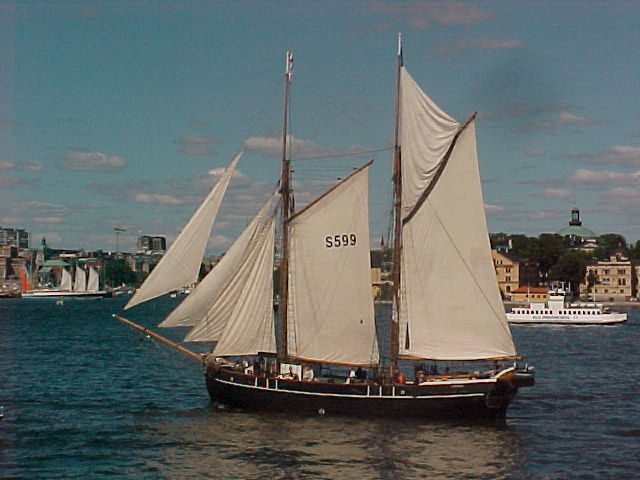The image captures a detailed side view of a sailboat with a sleek black body and large, white sails of various triangular shapes. Prominently displayed on the middle sail is the inscription "S 599." The boat is equipped with wooden masts and stakes that support the sails, including a prominent, long wooden pole at the front. The sailboat glides through a deep dark aquamarine ocean, reflecting its stark sails on the water's surface. In the background, the scenery includes more boats, a shoreline dotted with buildings, a green structure, and trees, all under a cloudy, dull, blue sky. The setting appears to be a bay, captured during the day.